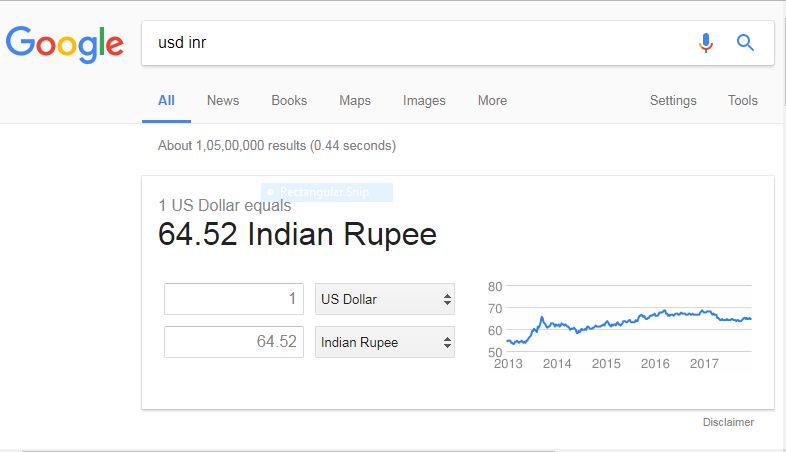This image is a screenshot of a Google search conducted on a computer, displaying the exchange rate between the U.S. dollar (USD) and the Indian rupee (INR). In the upper left corner of the browser, the colorful Google logo is prominently displayed. Adjacent to the logo, there is a long, white search box containing the query "USD INR." 

To the right of the search box, there are recognizable icons: a microphone symbol and a blue magnifying glass symbol indicating the search action. Below the search box, there is a horizontal menu bar with several categories: "All," "News," "Books," "Maps," "Images," "More," "Settings," and "Tools." Currently, the "All" category is selected, highlighted in blue with an underline, while the remaining categories are displayed in gray text.

Below the menu bar, Google indicates the number of search results available, stated as "About 1 billion results," alongside the search completion time, ".44 seconds." 

Centrally positioned on the page is a white information box displaying the current exchange rate: "1 U.S. dollar equals 65.52 Indian rupees," with the text presented in black. Below this, there is an input section where users can enter different amounts for conversion. An example provided shows "1" in the U.S. dollar field, translating to "64.52" in the Indian rupee field, with a labeled dropdown menu indicating the respective currencies.

In the bottom right corner of the screenshot, a small graph charts the historical exchange rate trend between the U.S. dollar and the Indian rupee from 2013 to 2017, depicted with a blue line that shows a slight upward trajectory, indicating a gradual increase in the value over time.